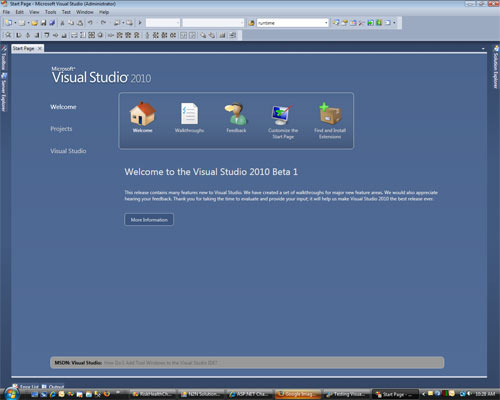The image appears to be a zoomed-in and somewhat blurry screenshot of a section of a website displaying an older interface of Microsoft Visual Studio 2010. Here's a detailed description:

The top part of the website features a gray navigation area. When zoomed in, the text becomes blurry, but it appears to include the words "star page" in black alongside "Microsoft". There are several menu options possibly labeled "File", "View", "Tools", "Text", "Windows", and "Help". Icons visible include a floppy disk symbol for "Save" and a gray arrow pointing left, likely for the "Undo" function. Additionally, there are three rectangular text input boxes, with something typed into the last one, but the text is indistinct and blurry.

The main background of the document displays a blue color. In white text, it says "Microsoft Visual Studio 2010," followed by "Welcome Projects View Visual Studio." Below this, there is an image of a beige and brown house. There is also a white piece of paper, but the text on it is unreadable. Another line reads "Feedback" adjacent to an illustration of a person in a green shirt. A blue computer monitor icon is present but the accompanying text is unclear. There's a cardboard box with a green plus sign, again, with illegible text underneath. The bottom of the image states, "Welcome to the Visual Studio 2010 Beta 1." The description also mentions two white lines that might represent text or font lines, but the content is not visible.